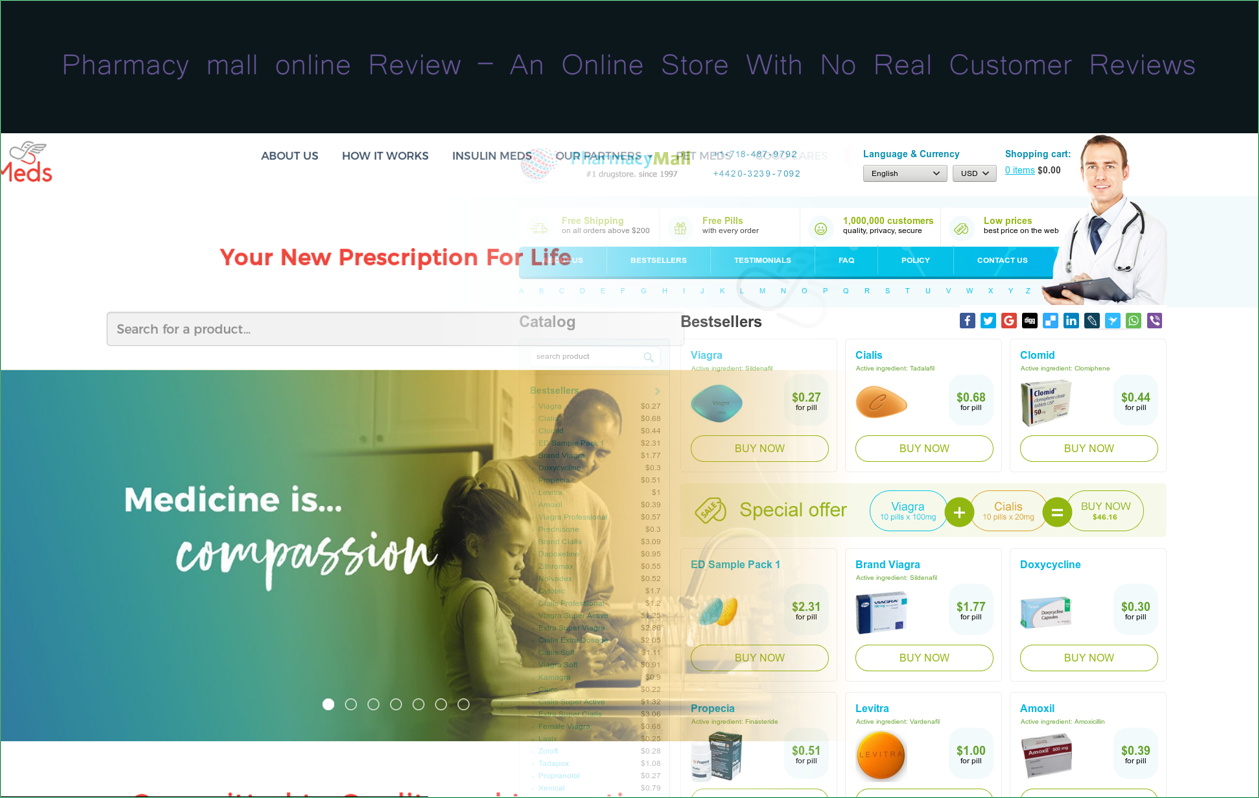This image is a partial screenshot of a pharmacy website. At the top, there is a black banner with purple text that reads, "Pharmacy Mail Online Review - An online store with no real customer reviews." The captured portion of the website shows the right side of the page, with the left side partially cut off. 

On the visible part of the website, there's a logo that includes the word "meds" in red, accompanied by an illustration of a capsule with wings flying above the text. Further down, a bold red text advertises, "This is your new prescription for life."

In the center of the image, there is a photograph of a doctor, visible from the waist up, wearing a white coat and a stethoscope around his neck. He is a white male with brown hair. The website's background is predominantly white or light-colored.

Below the doctor’s image, various medications are displayed, including a blue Viagra pill, an orange Cialis pill, and a box of Clomid. These medications are listed side by side in three columns, each shown with a name and price. For instance, Cialis is priced at 68 cents per pill. The overall feel of the website casts doubt on its legitimacy, as suggested by the banner text at the top.